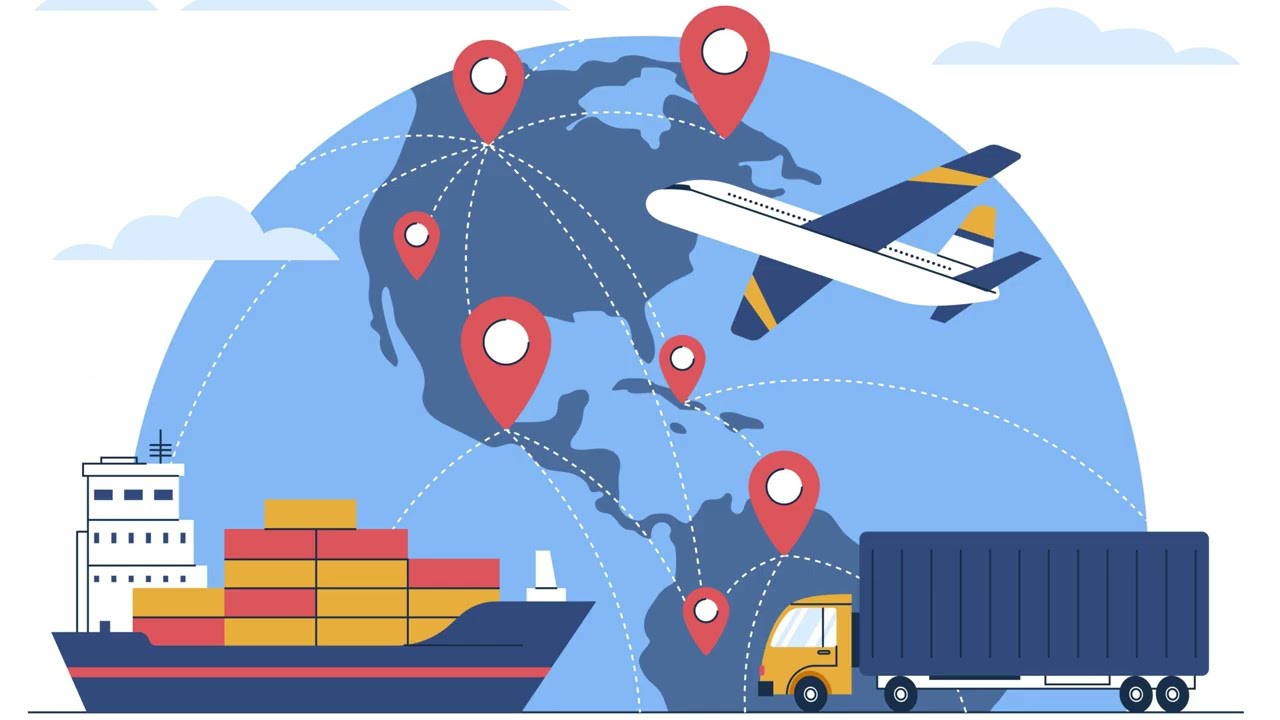This cartoon-style illustration from a logistics company is an eye-catching depiction of global transport. Dominating the image is a large, blue-tinted globe showcasing North and South America, with the land in dark blue and the water in light blue. The globe is intersected by white dotted lines that trace curved paths between red pinpoint markers, symbolizing key destinations and travel routes across the world. Floating above the globe are light blue clouds, adding to the whimsical feel of the image. Encircling the globe are three main forms of transport: a white airplane with blue and yellow wings to the right, a blue semi-truck with a yellow cab at the bottom right, and a dark blue cargo ship with a red stripe, stacked high with yellow and red shipping crates, to the bottom left. The various modes of transport signify the modern efficiency and multiple options available for global shipping. The cool blue tones and the inclusion of familiar geographic and logistical icons effectively illustrate the speed and ease of present-day international transportation.